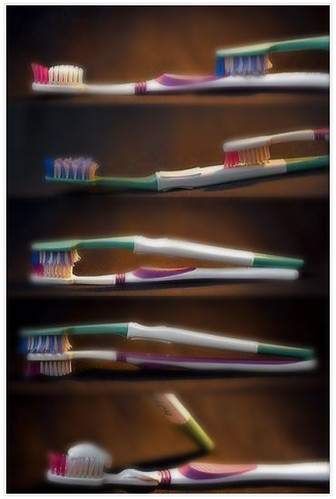The image is a detailed artistic representation of toothbrushes arranged to mimic various positions. It consists of a series of five scenes or 'shelves,' each depicting different interactions between the toothbrushes:

1. On the first shelf, a pink toothbrush lies on its back while a green toothbrush touches its lower end.
2. The second shelf shows the green toothbrush lying down with a red toothbrush positioned over its lower end.
3. The third shelf features the pink and green toothbrushes touching bristle-to-bristle, arranged with the green toothbrush on top and the pink one below.
4. On the fourth shelf, the pink toothbrush lies face down on the floor with its bristles touching the floor, while the green toothbrush is positioned above it, their bristles almost making contact with what appears to be the 'neck' of the pink brush.
5. The final shelf depicts the pink toothbrush lying down with toothpaste spread halfway from its center. The green toothbrush hovers above it, partially visible.

This tableau comprises various colored toothbrushes, including red, pink, green, and white, arranged in intricate and suggestive compositions.